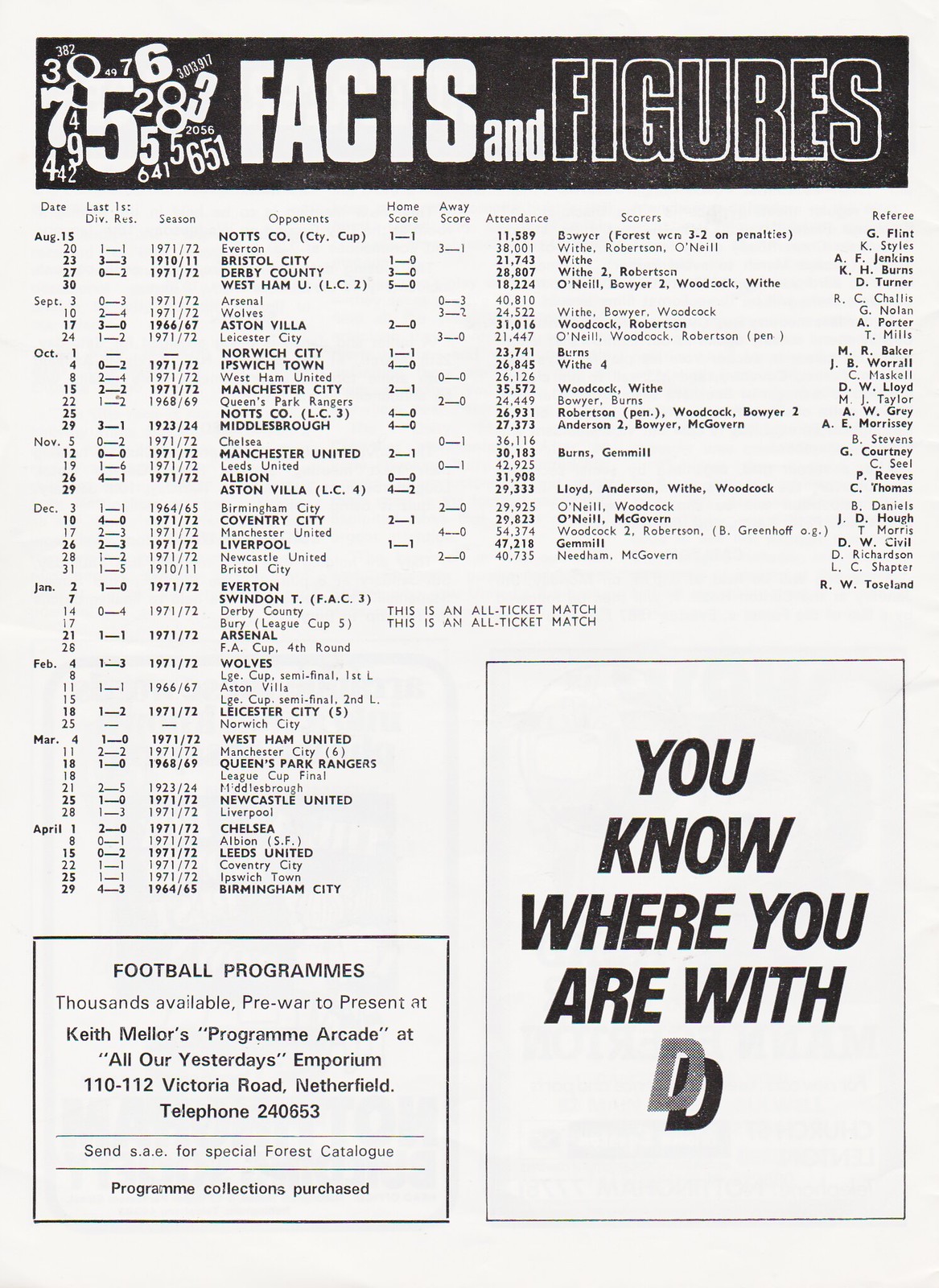This image is a detailed scan of a magazine page for European football (soccer) enthusiasts, featuring an eye-catching banner at the top that reads "FACTS and FIGURES." The word "FACTS" appears in white text, while "FIGURES" is highlighted black with a white outline, set against a dark background teeming with floating numbers. Directly underneath, the page presents a comprehensive list of teams such as Bristol City and Manchester City, with detailed scoring information for each match, including home and away scores, attendance figures, and opponent details. The page is densely packed with statistics, using small fonts to present the data clearly. In the bottom right corner, there's an advertisement stating, "Football programs thousands available pre-war to present at Keith Miller's Program Arcade at All Our Yesterdays Emporium, 110 to 112 Victoria Road, Netherfield, telephone 240653. Send SAE for special force catalog. Program collections purchased." Adjacent to this, a rectangular box contains the slogan "You know where you are with" followed by a 3D floating letter 'D' with a prominent drop-down shadow, serving as an additional advertisement. Overall, the page is a treasure trove of historical and statistical football information, blending data and advertisements seamlessly.